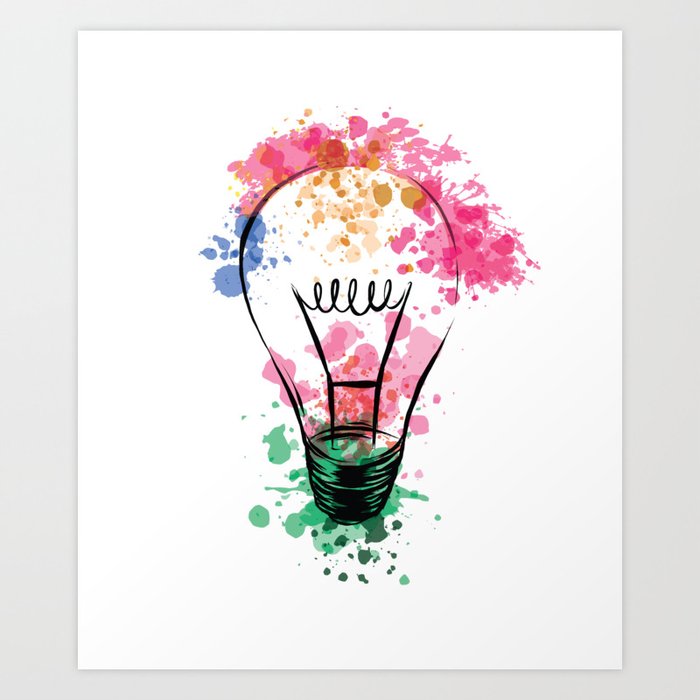The image features a detailed painting of an old-fashioned filament light bulb, centrally placed on a white canvas. The bulb has a glass dome and a black coil filament inside, with a screw-in holder at its base. The artwork, done in a stylus-like flatter art style, is highlighted by an intricate black sketch outline. Surrounding the bulb are splashes of vibrant watercolors: green hues near the holder, with blue, pink, and a hint of yellow splattered around the upper areas of the bulb. The background behind the canvas is a subtle, light gray, adding a minimalist contrast to the vivid artwork. There's no text within the piece, and the design evokes the feel of contemporary art that one might find displayed in a modern gallery.